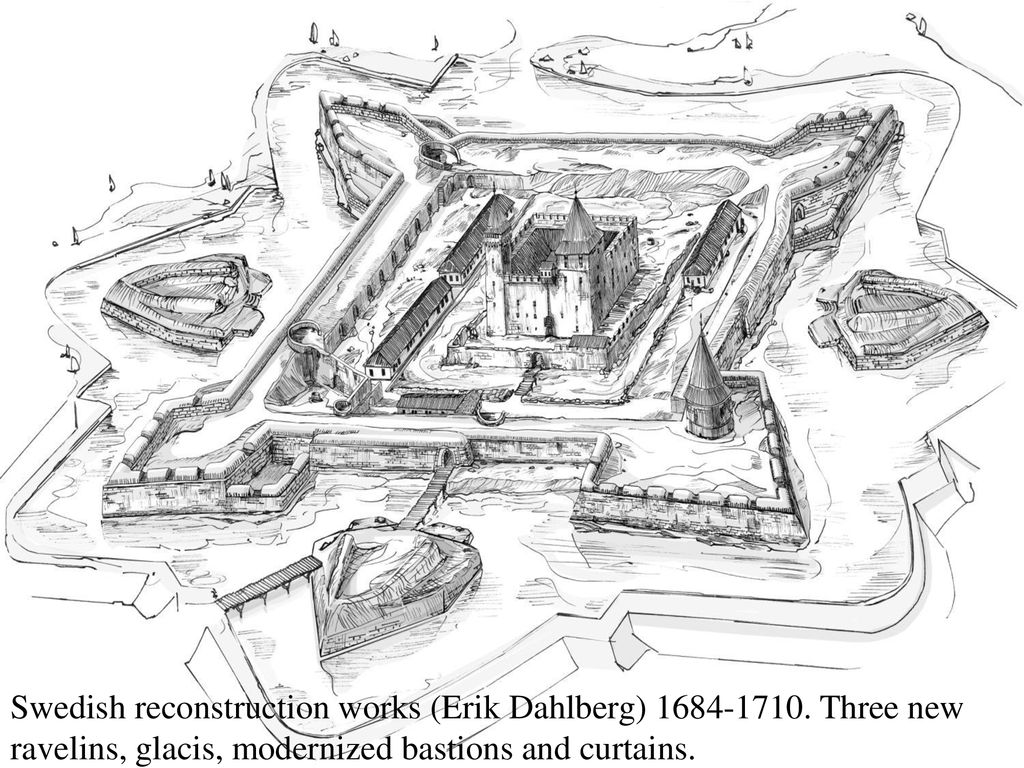This historical drawing, created by Eric Dahlberg between 1684 and 1710, showcases Swedish reconstruction works of a castle fortress. It features a detailed schematic layout for enhancing the defensive structures of the fortress. The plan includes three new ravelins, glasses, modernized bastions, and curtains. The black-and-white illustration depicts a star-shaped moat with seven pointed defenses. The moat, indicated by shaded water, surrounds the fortress and includes parapets, small bunkers, and drawbridges connecting to the stronghold. Inside the heavily fortified rectangular perimeter, with sharply pointed geometric corners, lie inner castle walls, various buildings, and homesteads, culminating in a central castle. The intricate details, such as gates and bridges, emphasize the comprehensive defensive upgrades proposed in this period-specific reconstruction blueprint.